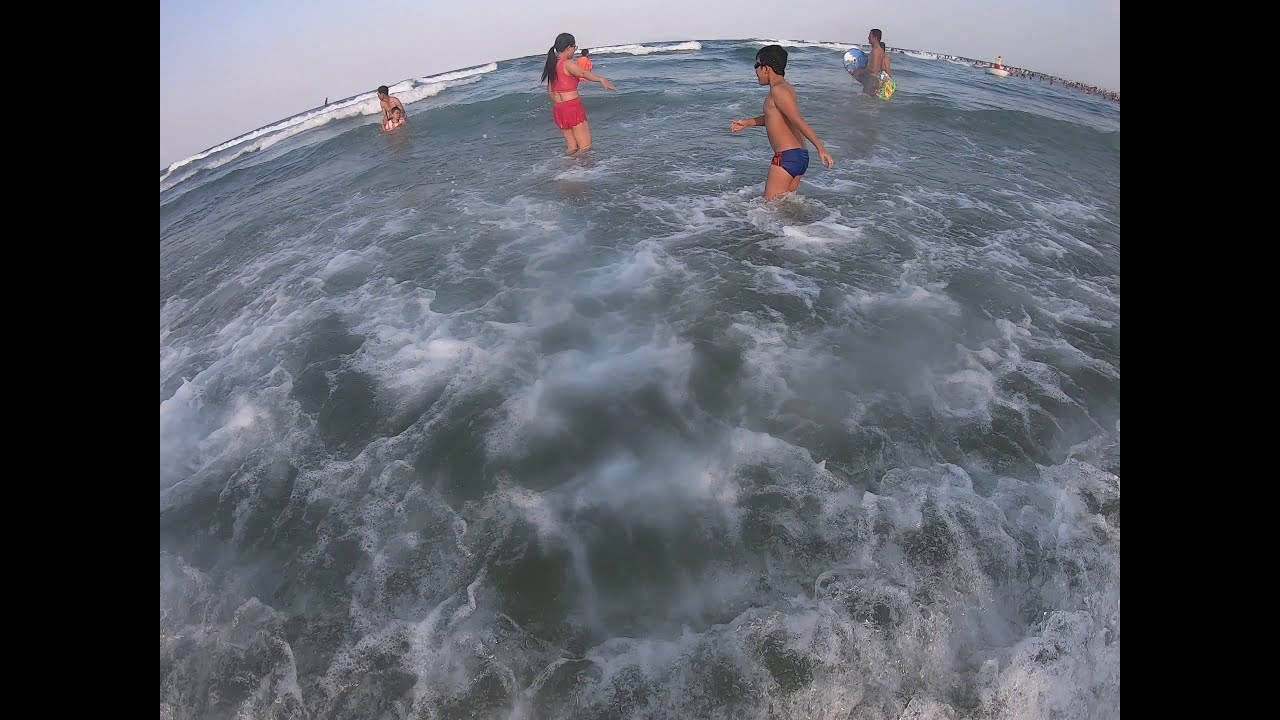A vivid photograph captures a lively scene at the beach, showcasing individuals frolicking in the ocean. The seawater appears black and white, the white hue resulting from the bubbles and foam created by the breaking waves, and the water itself has a black or grayish tint in parts. Dominating the foreground is a girl with dark, long hair tied in a ponytail. She stands knee-deep in the foamy sea, wearing a red bathing suit with her arms outstretched. Close by, a boy in blue swim trunks and sunglasses wades in the water, which reaches up to his thighs. Behind them, about four more people are seen enjoying the waves that roll in from the distance. Overhead, the sky is a clear, light blue, enhancing the bright and cheerful atmosphere of the scene. The photograph, taken in fisheye mode, adds a unique curvature to the image, further accentuated by vertical black strips on both the left and right sides. This perspective makes everything appear rounded, as if viewing a small part of a spherical world.